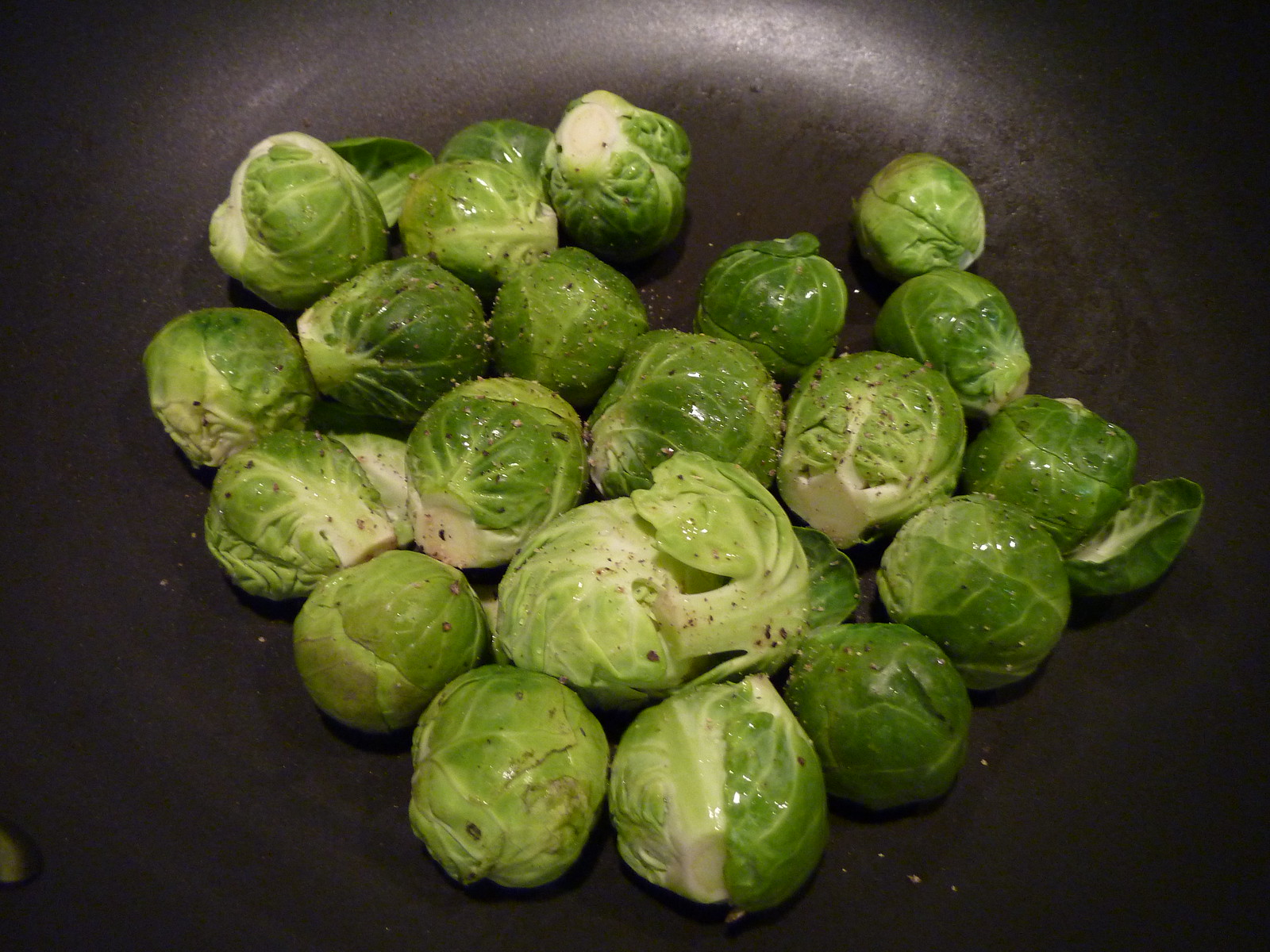This photograph captures a black non-stick pan with a satiny finish, featuring traces of charring and a slightly greasy look in the center. Inside the pan are numerous whole brussels sprouts, exhibiting a dark green hue with lighter areas around the stem and white specks scattered on their leafy, ridged exteriors. The brussels sprouts appear to be lightly seasoned with pepper and salt, and though they seem to be prepped with some oil, they haven't yet begun to cook, as evidenced by the lack of typical charring. The detailed leaves and veins of the sprouts are clearly visible, adding texture to the scene. A stud visible in the bottom left corner likely secures the handle to the base of the pan, emphasizing the practical yet understated nature of the kitchenware.